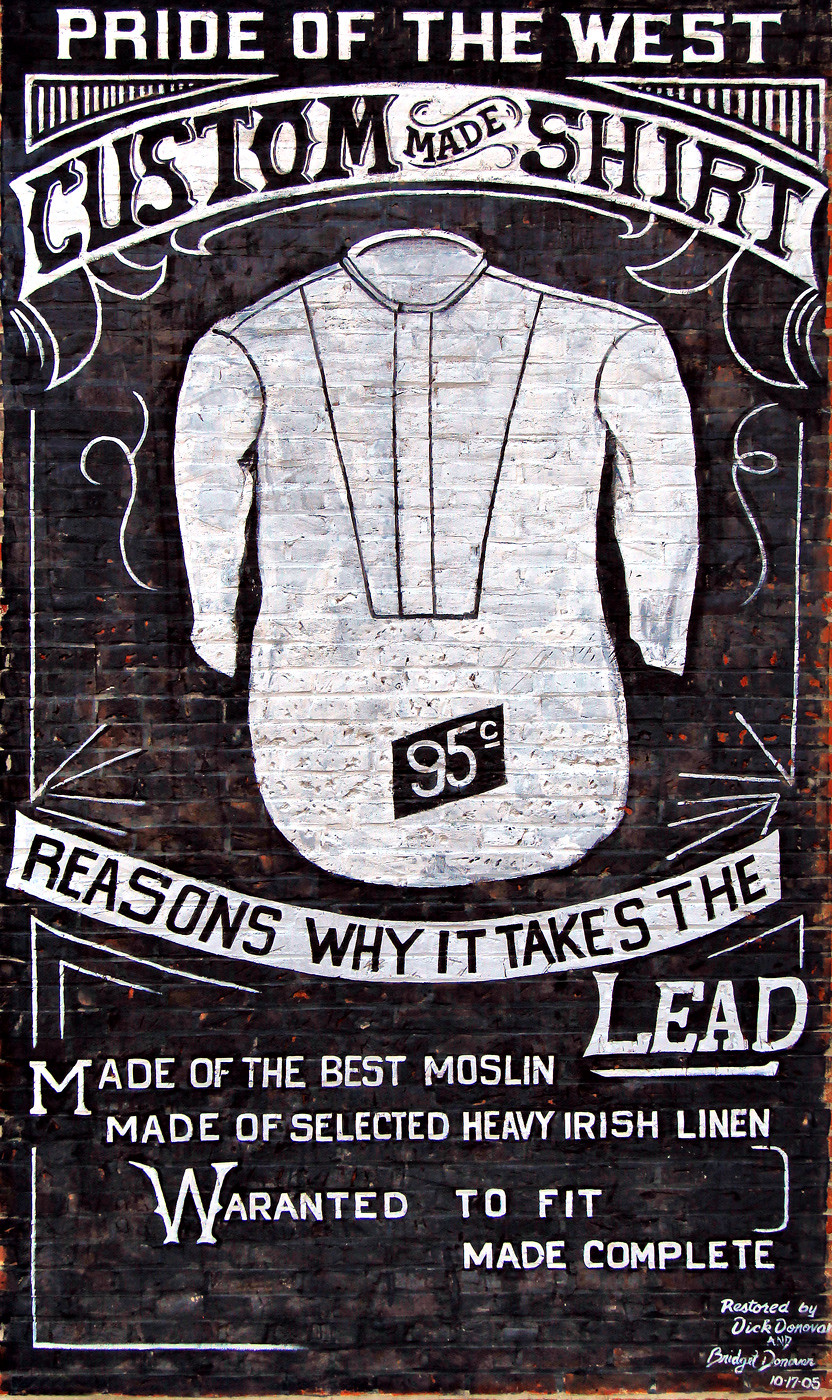The image depicts a detailed graphic art piece on a black brick wall, primarily using black and white tones. At the top of the graphic, the text "Pride of the West, Custom-Made Shirt" is prominently displayed. Below this, there is a depiction of a long-sleeve button-up shirt, priced at 95 cents. A banner across the image states, "Reasons why it takes the lead." Further descriptive text reads, "Made of the best muslin, made of selected heavy Irish linen, warranted to fit made complete." The graphic concludes with the restoration details at the lower right, stating, "Restored by Dick Donovan and Bridget Donovan, October 1705."